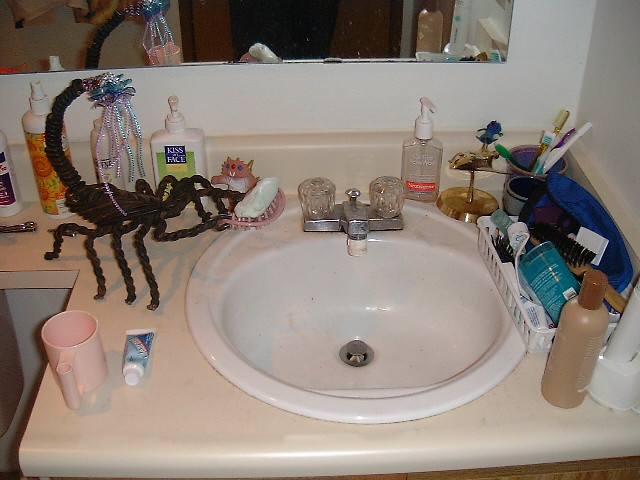The image is a snapshot taken in someone's bathroom, showcasing a whimsical mix of practicality and humor. The focal point is a standard white, possibly porcelain, round sink set into a basic pale tan Formica countertop with a rounded front edge. To the left, the counter extends narrowly over a toilet, reminiscent of older bathroom designs. 

A frameless, wall-mounted mirror, secured with clips, reflects the simple white walls. Positioned above the sink is a cheap two-handle chrome faucet. The counter is cluttered with various items, adding to the lived-in charm.

On the right side of the counter sits a bottle that could be either hand sanitizer or pump soap. Next to it, a brass stand poses a mystery; behind it rests a stoneware cup crammed with toothbrushes, making its purpose unclear. In front of the toothbrush cup is another small cup that appears empty.

A white, low plastic organizing bin or tray holds an array of daily essentials including deodorant, a cosmetic bag, a hairbrush, and tubes of toothpaste or mascara. Nearby, in the right corner, a corded rechargeable toothbrush and a possibly lotion-filled bottle find their place.

Dominating the left side of the sink is a quirky, oversized scorpion sculpture made from twisted black wire. The scorpion features a festive, glittery bow hanging from its elevated stinger tail and holds a nubby soap dish in its pincers, cleverly positioned to allow the soap to drip and dry over the sink. 

Against the backsplash is a "Kiss My Face" pump bottle of cleanser or lotion, flanked by what appears to be a deranged cat or chipmunk figurine, adding to the eclectic mix. A spritz bottle, potentially for room or body spray, stands to the left of the lotion.

This humorous and chaotic array is highlighted by the striking black wire scorpion, making it the key visual element of the photo.